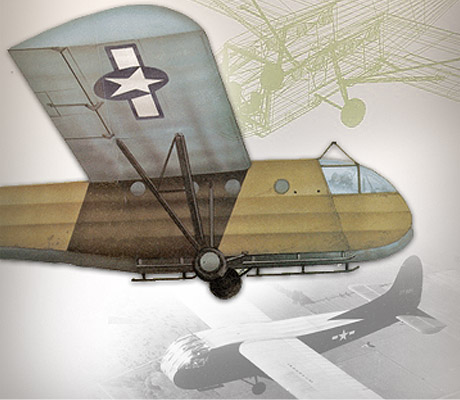This composite image showcases three views of a World War II-era glider plane, used during the Normandy invasion to transport soldiers behind enemy lines. The primary focus is a meticulously detailed drawing of the brown, old-fashioned aircraft with silver wings adorned with a distinct blue and white military emblem. The fuselage features a light brown color, punctuated by a dark brown stripe beneath the wings. The plane’s structure includes straight wings and skids, with both the clear, rounded cockpit windows and small circular windows indicating its boxy design. A notable feature is the hook atop the cockpit, which was used for towing the glider.

Beneath this detailed drawing is a vintage black and white photograph of the same plane in flight over a field, oriented leftward and slightly downward, providing context to its real-world operation. Above the main drawing, there is an x-ray view of the aircraft, showing its inner structure and beam framework. This portion of the image is rendered in gray-green tones on a light gray background, providing a technical perspective on the plane’s construction. The entire image is set against a subtle light gray backdrop, giving it a unified and cohesive appearance.